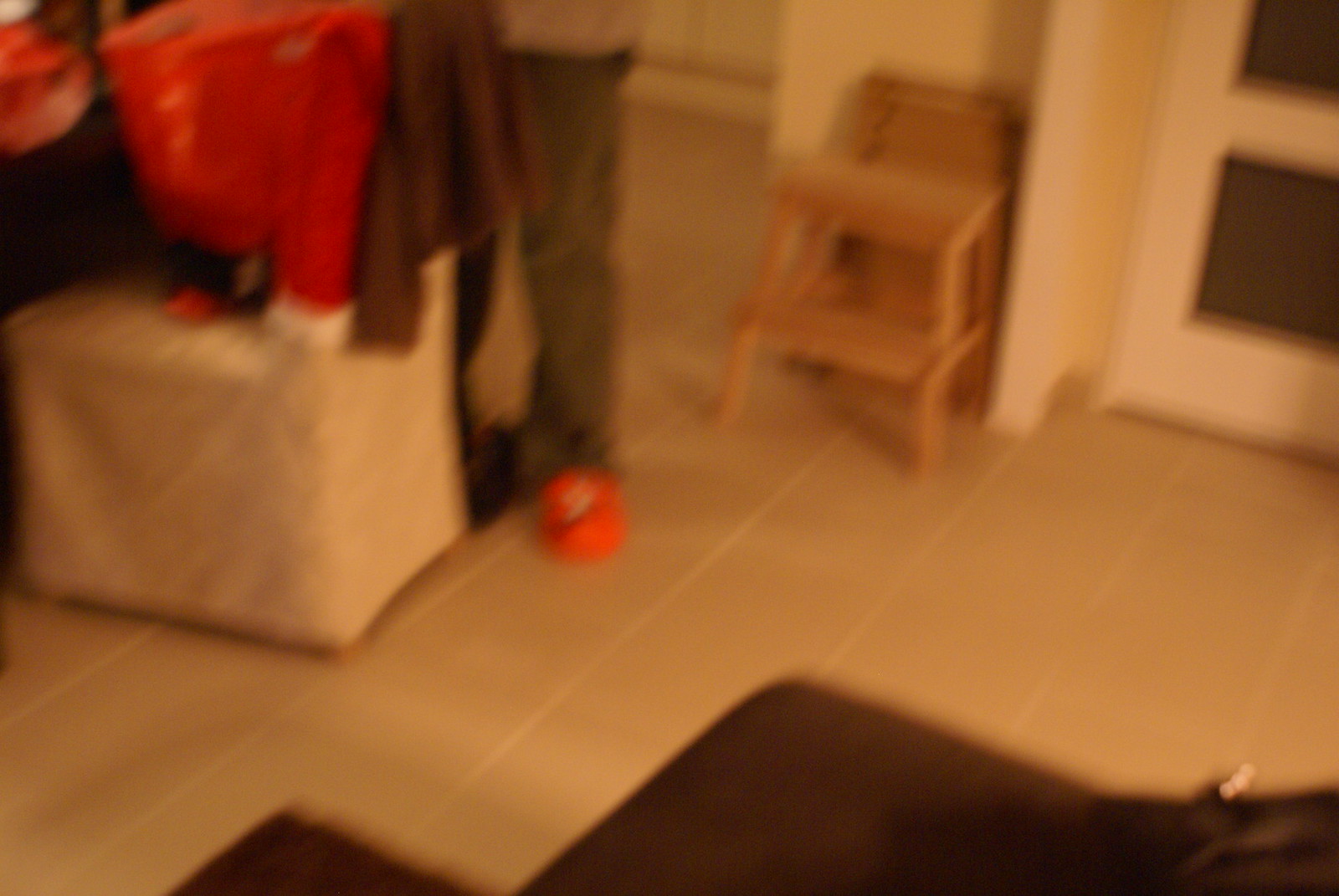This blurry photograph appears to have been taken inside someone’s home, likely during evening time as the lighting seems to emanate from lamps. The scene includes a grid-patterned tile floor and a light-colored wooden step stool, or perhaps a high chair. The bottom of the image is obscured by shadows. On the right, there’s a partial view of a door leading to another room. 

In the center, there’s a large white ottoman or hamper with a variety of items on top. A red plastic bag and several articles of clothing, including dark green and brown pieces, and a red garment with white trim reminiscent of a Santa outfit are visible. There's also a person standing nearby, possibly engaged with the items, dressed in green corduroy pants and orange shoes. The back of a wooden chair draped with a festive chair cover in the style of a Santa hat is also visible. Overall, the room appears cluttered and the photograph’s low resolution makes identifying specific objects challenging.